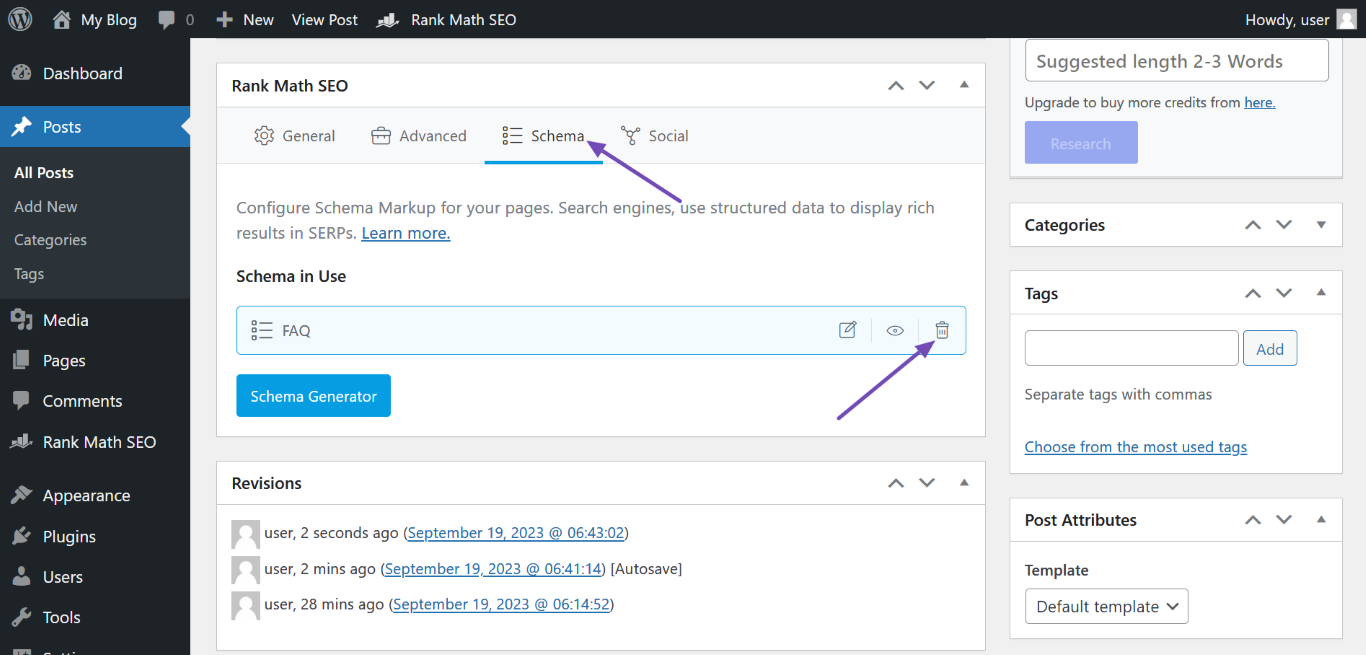Screenshot of a user's blog management dashboard interface displaying the "My Blog" header. The screenshot features a navigation bar on the left side where the "Posts" section is highlighted in a blue rectangle. Additional navigation options visible in the black sidebar include: All Posts, Add New, Categories, Tags, Media, Pages, Comments, Rank Math SEO, Appearance, Plugins, Users, and Tools. The bottom portion of the sidebar is partially cut off.

In the main content area, Rank Math SEO settings are displayed with tabs for General, Advanced, Schema, and Social. A prominent purple arrow points to the "Schema" tab, indicating it's the current focus. Below, another purple or red arrow points towards a trash can icon next to the label "FAQ" under the "Schema in Use" section. There is also a clickable blue button labeled "Schema Generator" to further interact with the settings.